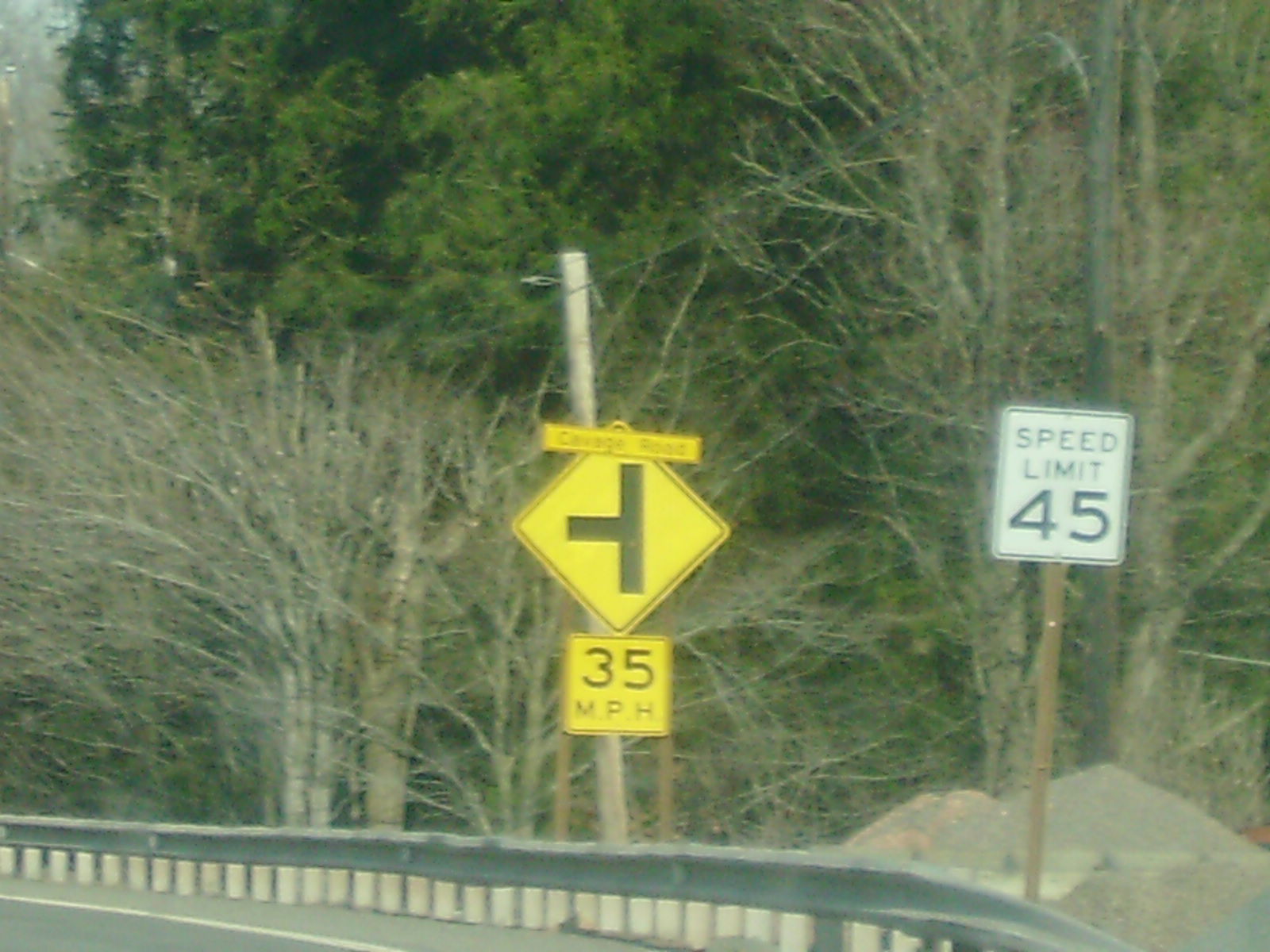This outdoor photograph captures a somewhat hazy, poor-quality image of a roadside scene. The foreground features a small area of road with a white line on the bottom left corner, bordered by a metal guardrail. Two road signs are prominently displayed on poles adjacent to the guardrail. The first, on the far right, is a white rectangular speed limit sign indicating 45 miles per hour, with a black border. To its left, a yellow diamond-shaped sign displays a T-junction symbol, and beneath it, a square sign reads 35 miles per hour. Above the top sign is a partially visible name of the road, though only the word "road" can be discerned due to the blurriness. Behind the guardrail, a wooded area emerges, with bare, grayish trees in the foreground that appear almost dead, their branches stripped of leaves. In contrast, bushy green trees populate the distant background, adding a touch of foliage to the scene.